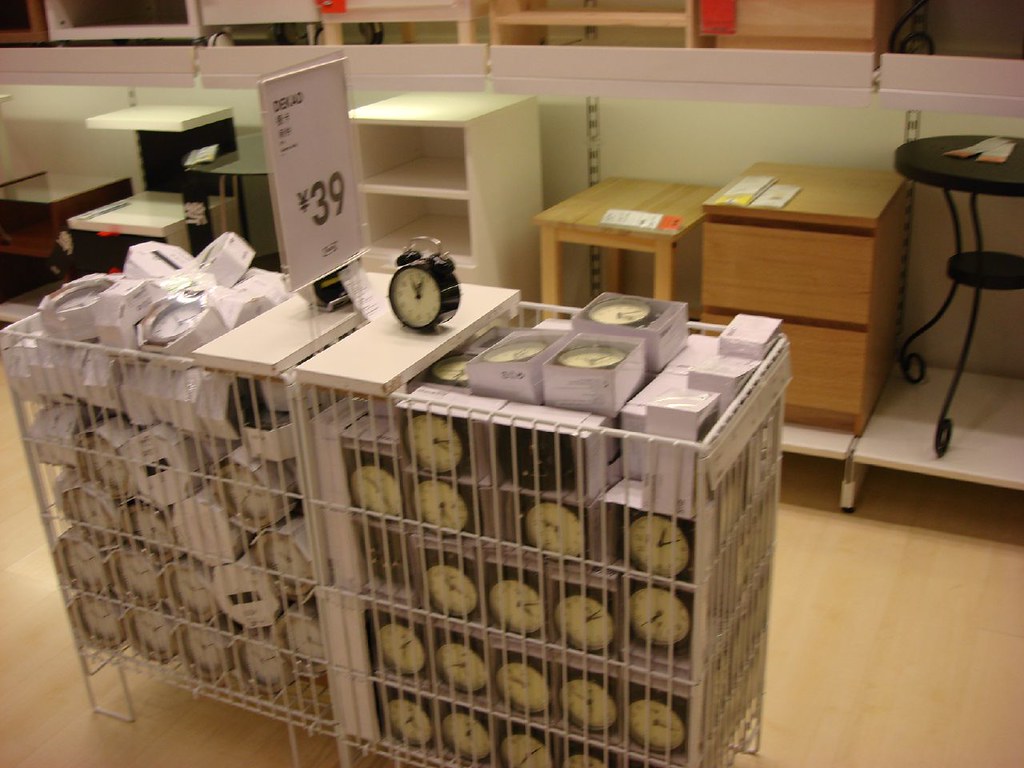In a furniture store filled with various office essentials such as rolling file cabinets, small tables, and shelves, there is a prominent display that draws attention. This display features several cages containing neatly boxed alarm clocks. The clocks come in two colors: black and white, with each color organized on opposite sides. These analog alarm clocks, equipped with traditional bells on top, are presented in simplistic white boxes that are open-ended, allowing customers to see the product's design. The clock faces exhibit a yellowish hue, possibly indicating a glow-in-the-dark feature. Notably, these clocks are priced at what appears to be $39, based on the displayed signage which includes an oriental currency figure, suggesting a translation or cultural context. The price seems unexpectedly high for such items, adding an element of curiosity to the display.